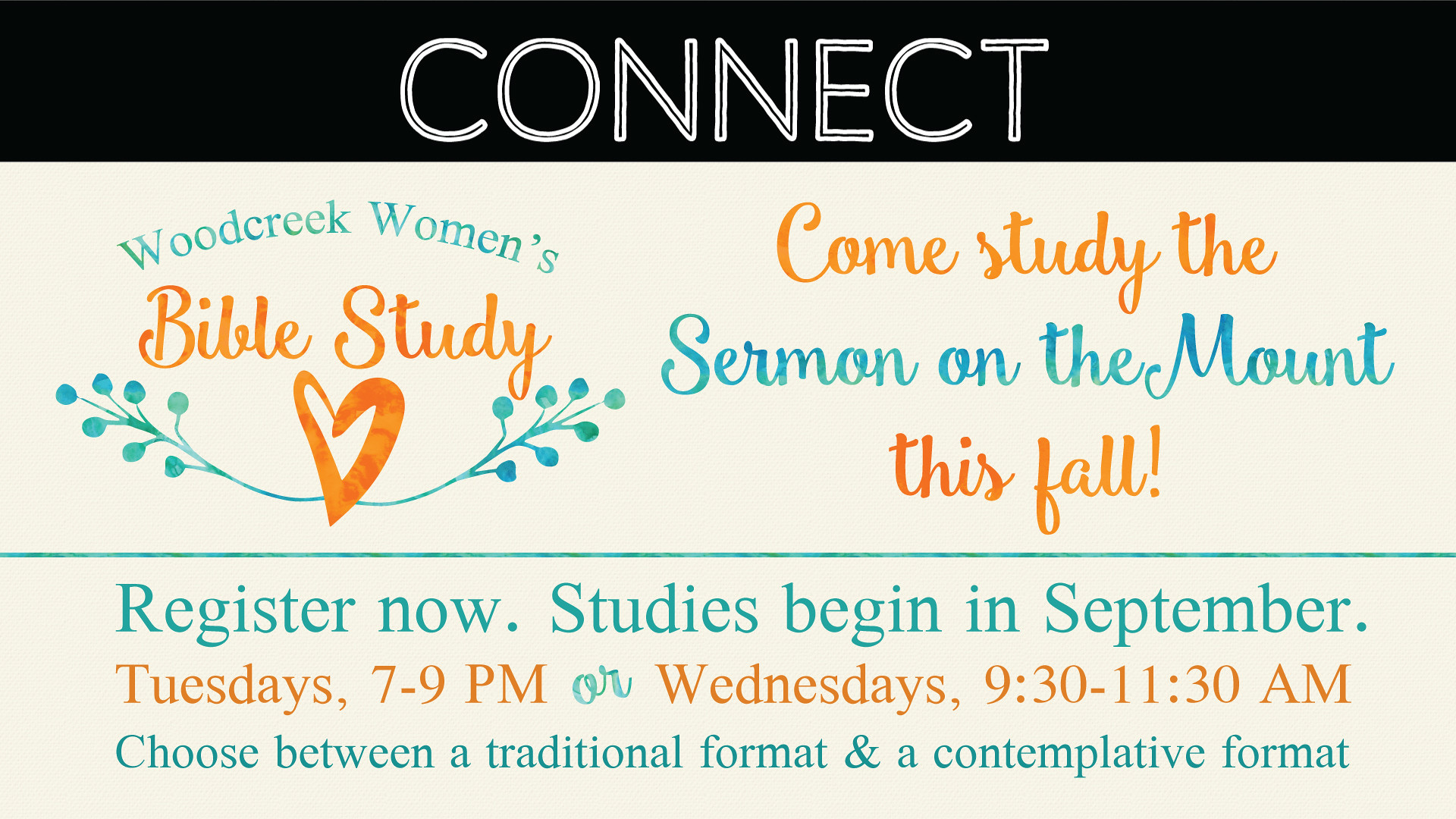The image is an advertisement for an upcoming event at Wood Creek Church, focusing on a women's Bible study. At the top, the word "Connect" appears in white text against a black background. Below it, on a beige background, "Wood Creek Women's Bible Study" is prominently displayed, with "Wood Creek Women's" in blue and "Bible Study" in orange. Underneath, a small orange heart is flanked by green-blue leafy branches. The main text invites viewers to "Come study the Sermon on the Mount this fall," with "Come study" in orange and the rest in green. A green line separates this portion from the registration details below. The line "Register now. Studies begin in September" is written in blue. Participants can choose between meeting on Tuesdays from 7 to 9 p.m. or Wednesdays from 9:30 to 11:30 a.m., with the times highlighted in orange. The final line offers a choice between a traditional or a contemplative format, presented in blue. The clean layout and balanced color scheme make the information easy to read and visually appealing.